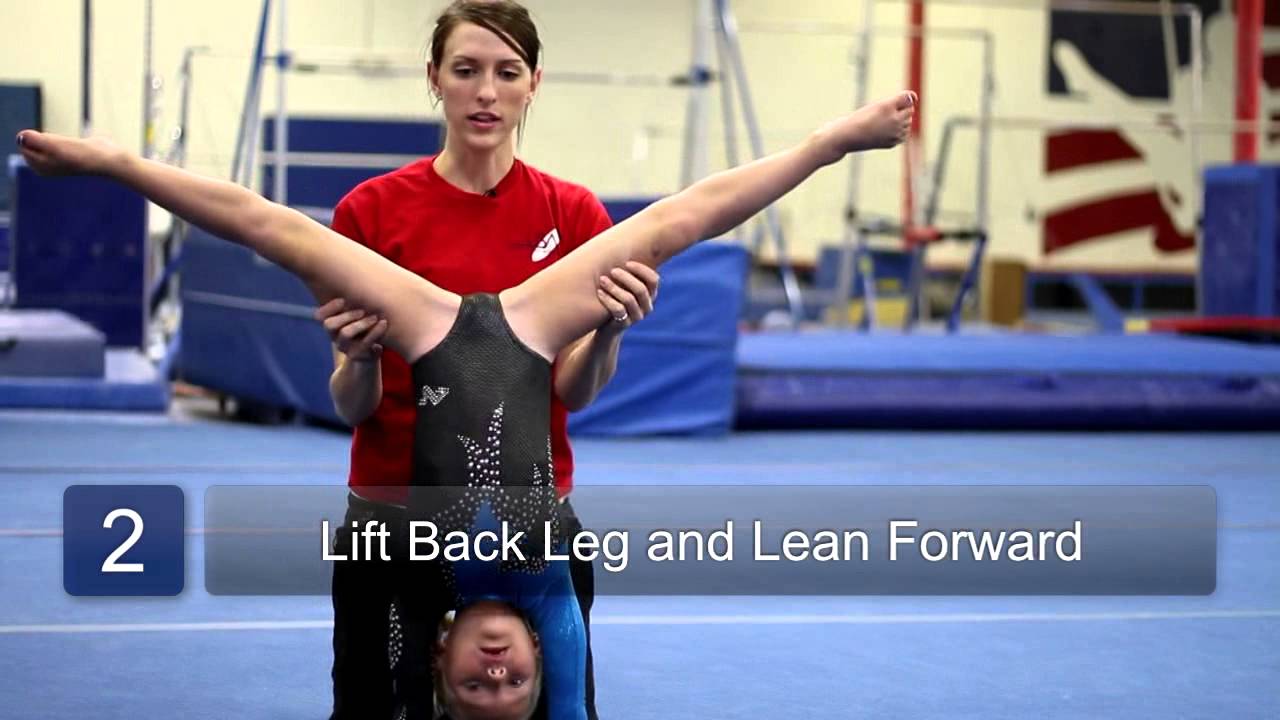The photograph captures an instructional moment inside a gymnastics facility. The foreground features a young girl, likely around 7 or 8 years old, executing a handstand split in a blue and black leotard adorned with rhinestones. Her legs are spread apart as her instructor, a woman with dark brown hair tied back and dressed in a red t-shirt and black pants, supports her by holding her thighs. The background reveals a typical gym setup with blue cushioned mats scattered across the floor and various gymnastics equipment, including the uneven bars, slightly blurred in the distance. A noticeable number 2 is displayed with the text "lift back leg and lean forward," suggesting this scene might be part of an educational program or instructional material. The walls of the room are white, enhancing the visibility of the vibrant gym colors.